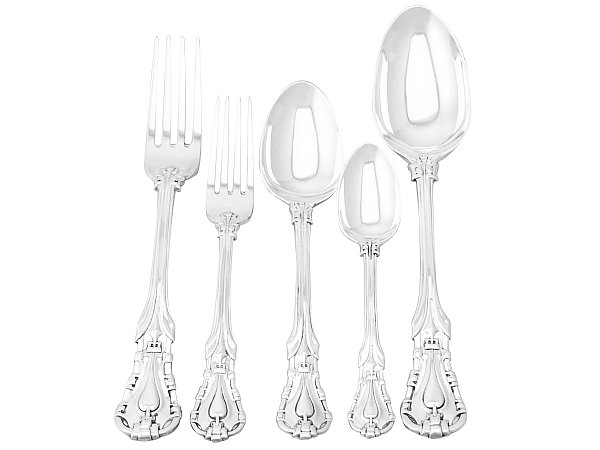This photorealistic image showcases a meticulously arranged set of silverware on a plain, white background under bright lighting, making the metal gleam with a silvery brilliance. The ornate design near the bottom of each piece features intricate curves and stylized motifs, adding a touch of sophistication to the set. From left to right, the lineup begins with a large dinner fork, its four tines pointing upwards. Next is a smaller salad fork, identical in design but shorter in stature. Following the forks is a medium-sized soup spoon, its smooth bowl oriented upwards. To the right of the soup spoon is a slightly smaller dessert spoon, and finally, at the far right, is a larger main course spoon, matching the height of the dinner fork but with a wider bowl. The precise arrangement and reflective nature of the silverware create an almost ethereal, clear appearance due to the intense brightness highlighting their polished surfaces.